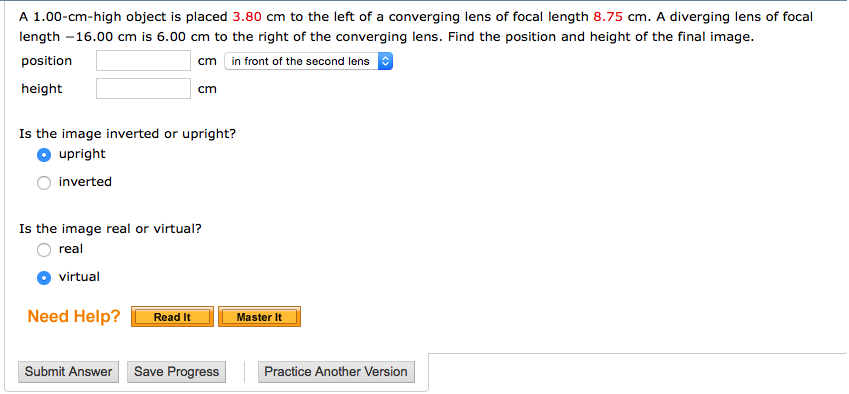Here is a cleaned-up and detailed caption for the described image:

---

The image features an all-white background with a thin black border running along the top and a thin gray border down the left side, extending horizontally about halfway, then ascending approximately an inch before crossing off to the right side. In the upper-left corner, there's a bold, but not overly prominent, black letter "A". Below this, in black text, it reads "1.00-CM-HI object is placed", followed by "3.80" in red, and back to black, "CM to the left of a converging lens, a focal length". Continuing in red, "8.75" is specified, then reverting to black, "CM." It mentions a "diverging lens, a focal length-16.0-CM" located "6.00-CM to the right of the converging lens." The sentence concludes with, "Find the position and height of the final image."

Directly below this narrative, the text "position" appears on the left, adjacent to a white, empty rectangle labeled "CM" on its right side. To the right of this rectangle is another white rectangle marked with "in black in front of the second lens" and accompanied by a blue square featuring upward and downward pointing white greater-than symbols.

Beneath this, the word "height" is situated on the left next to another rectangle, similarly labeled with "CM" on its outside. A small gap under the black lettering poses the question: "is the image inverted or upright?" Below this question, options for "upright" and "inverted" are presented. The "upright" option is to the left, paired with a blue circle, while the "inverted" option is next to a white circle with a gray border.

Further down, another question asks, "is the image real or virtual?" The options "real" and "virtual" are shown below, with "real" beside a white circle with a gray border and "virtual" indicated by a blue circle.

At the bottom, in orange text, the phrase "need help?" is followed by two adjacent orange tabs. The first tab reads "read it" in black, and the second tab reads "master it" in black. Finally, in the bottom-left corner, three gray tabs with black text are present, stating "submit answer," "save progress," and "practice another version" from left to right respectively.